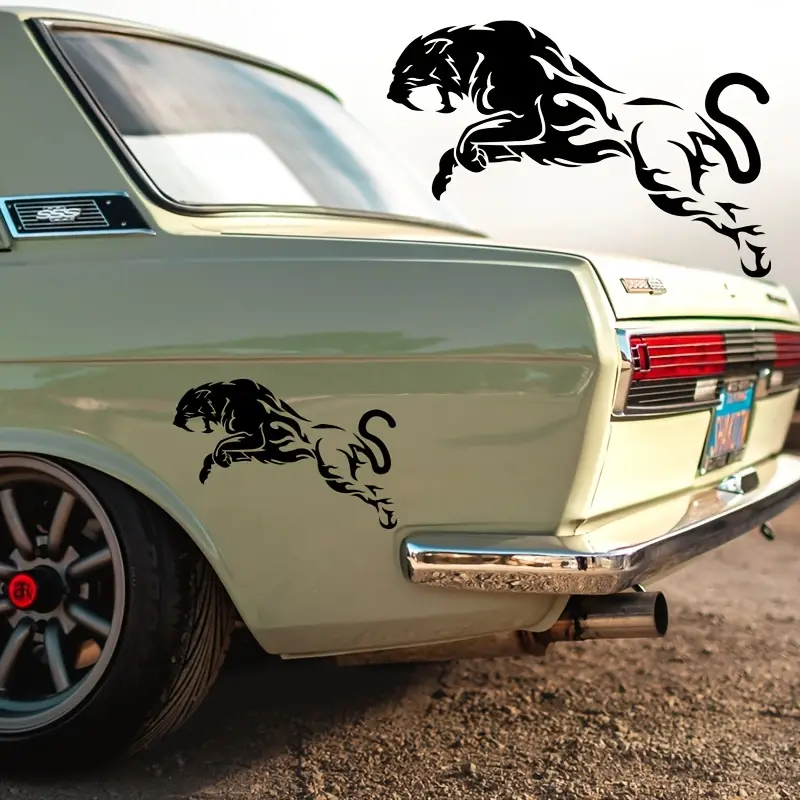This photograph showcases a meticulously remodeled vintage car, predominantly a yellowish-green sedan, situated on a dirt road. The back half of the car features distinctive details: a black decal of a pouncing feline, likely a mountain lion or puma, appearing both on the car and in a floating, more detailed rendition above it. The car's rear end boasts a chrome bumper and dual chrome exhausts, complemented by red taillights that stretch across the width of the vehicle. The rear window has a black "SSS" logo between the side windows and the rear windshield. The wheels are notable for their red hubs and spoked design. Additionally, a blue license plate with orange letters is visible, further emphasizing the car's vintage aesthetic.